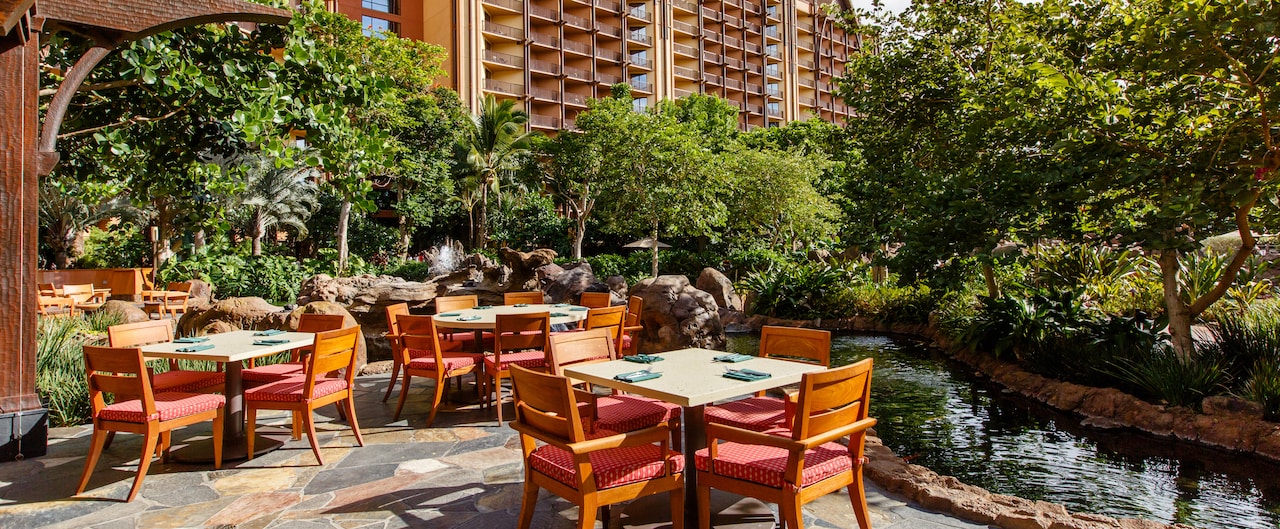This detailed photograph captures a sunny day at an outdoor patio of a restaurant, nestled beside a serene, artificially designed river that flows gracefully through a cityscape, surrounded by verdant trees on the right. The patio, featuring a charming stone or cobblestone floor, is set with several square tables each accompanied by four wooden chairs adorned with red cushions patterned with white dots. A single larger, round table occupies the center with similar chairs. Silverware is neatly arranged on the tables, ready for diners. In the background, a towering residential building, possibly a hotel, looms with numerous balconies. A dark wooden archway frames part of the scene on the left, adding an architectural touch to this picturesque urban oasis.